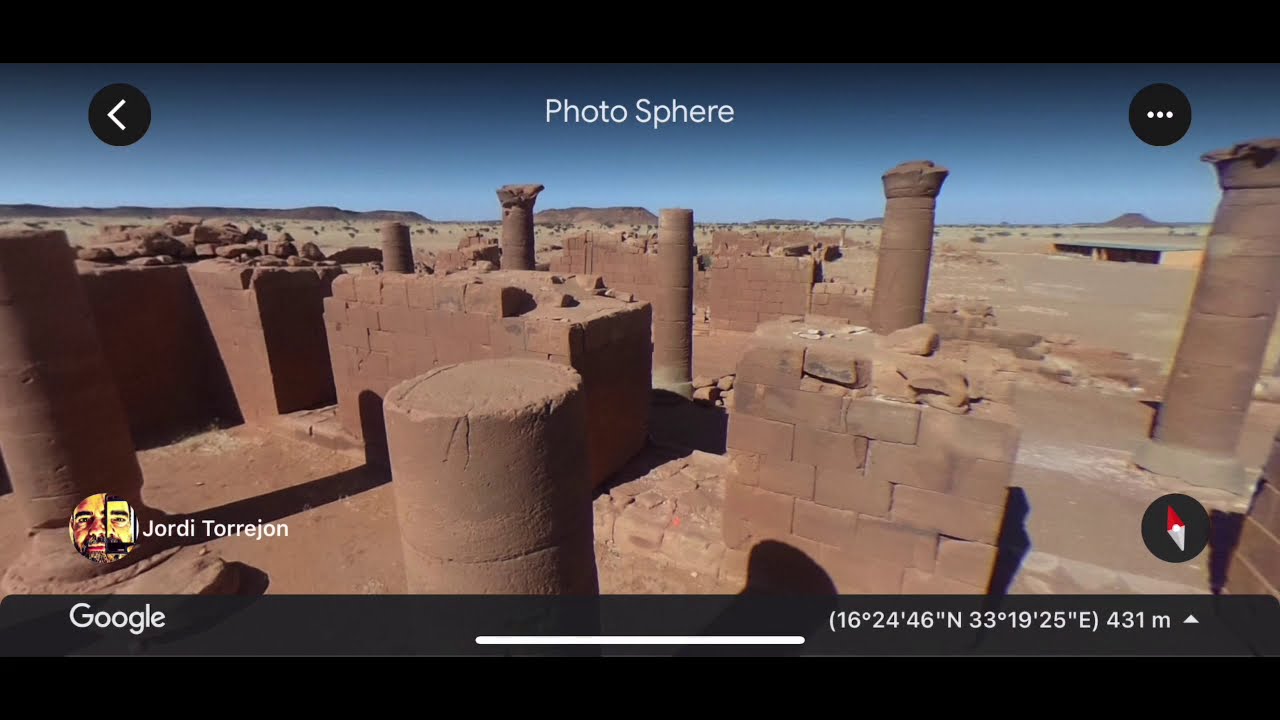The image is a Google Photosphere view capturing an ancient historic site situated in a desert. Dominated by light brown tones, the scene features a series of round columns and walls built from large rectangular bricks, suggesting the ruins of an old, possibly Egyptian or Greek, structure. The sky above is a clear light blue, stretching across the upper third of the image. At the top center, the word "photosphere" is displayed in white font. Towards the bottom, the Google interface appears with specific coordinates: 16°24'46" N, 33°19'25" E, along with an elevation of 431 meters and an up arrow. The bottom left corner showcases a circle with the user avatar of Jordi Torrijon, named as the photo's contributor. The bottom right corner features a compass for orientation. The entire image is framed with black letterbox bars at the top and bottom.